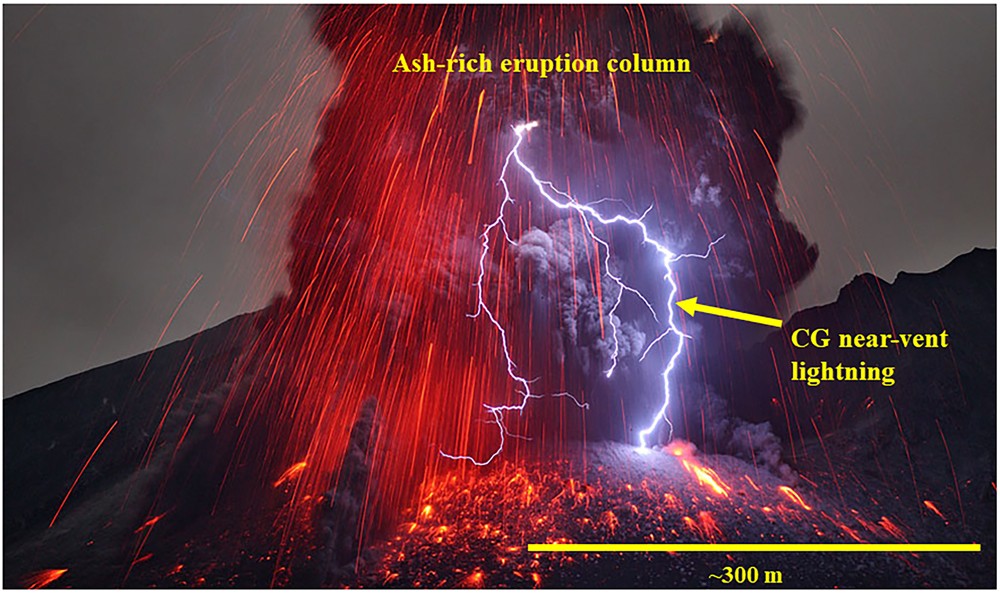This detailed photograph captures a dramatic, ash-rich volcanic eruption occurring during the evening. The top of the image features yellow text stating "Ash Rich Eruption Column," clearly identifying the event. Prominent in the scene, a massive dark eruption cloud dominates the sky, filled with red-hot volcanic material blasting upwards and cascading down. The center of the eruption is illuminated by an intense, bright blue and white lightning bolt, identified by a yellow arrow labeled "CG near vent lightning." This lightning, generated by the static electricity within the dense ash cloud, strikes toward the ground amidst the dark, foreboding clouds. Beneath the tumultuous scene, the magma and lava flow relentlessly, marked by a 300-meter measurement standard at the bottom of the image, providing scale to the viewer. The smoky gray background accentuates the fiery eruption and the chaotic beauty of nature's powerful forces on display.